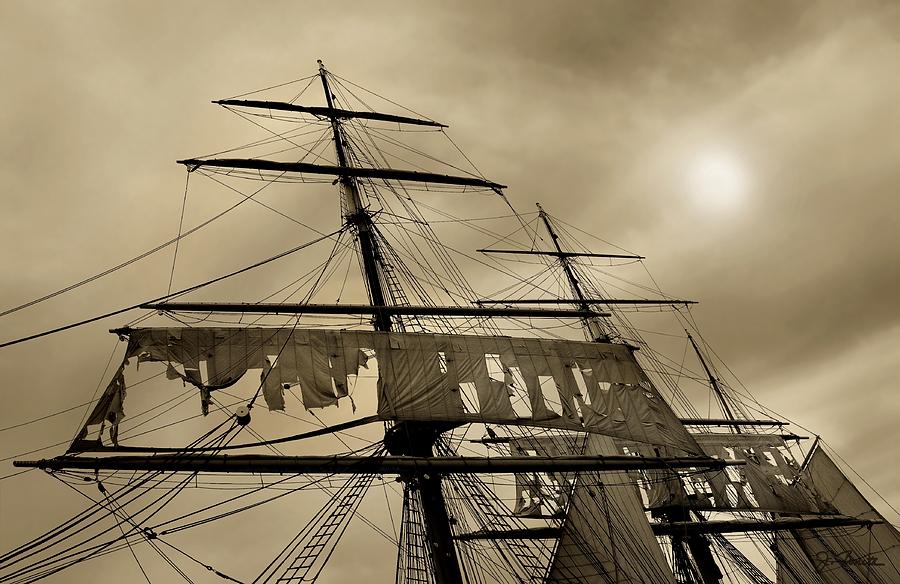This striking photograph portrays an aged, partially torn set of sails from a ship, reminiscent of those seen on pirate vessels in movies. Captured from a unique diagonal angle, the image reveals the sails rising upwards, outlined against a nearly monochromatic sky that darkens dramatically, almost suggesting a black-and-white scene. The sun can be glimpsed in the upper right corner, adding a stark contrast. The sails are depicted with intricate detail, showcasing the ropes, wooden structures, and frayed plastic components, though the ship's hull itself is not visible. Instead, the photograph focuses on the sails' base up through their towering heights, suggesting multiple sails, with at least one large and one small, and perhaps a third, indistinct in the composition. This evocative scene combines a sense of historical nostalgia with the raw texture of maritime wear and age.